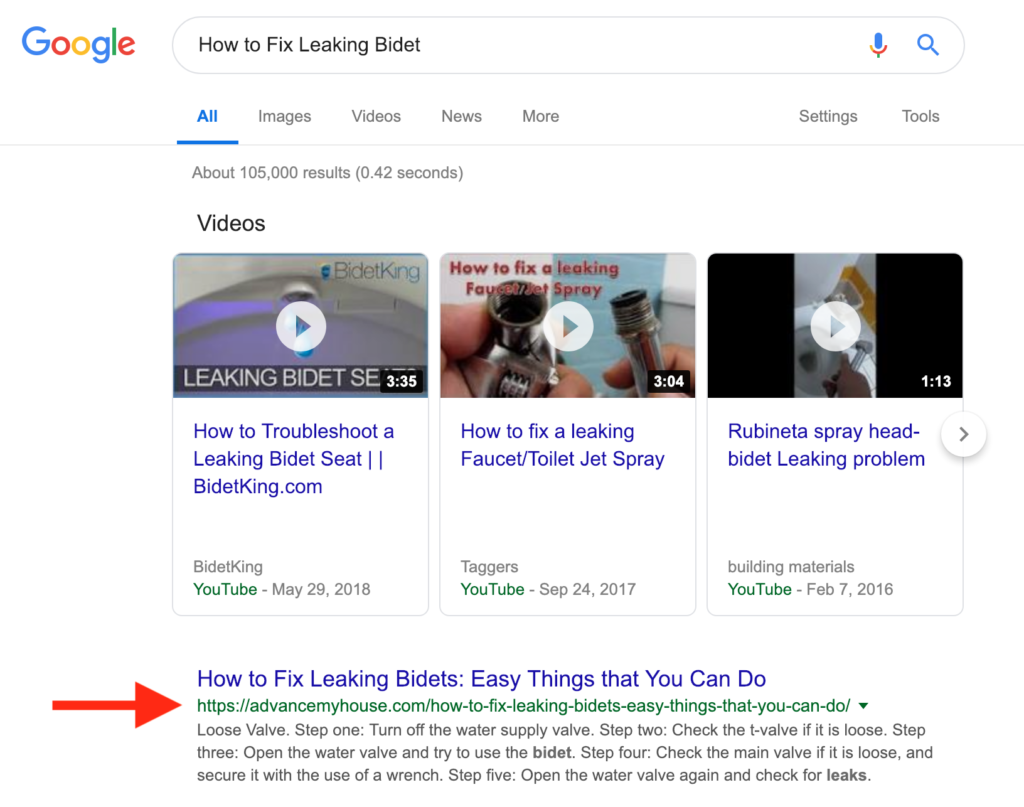The image depicts a Google search results page. At the top left, the familiar Google logo is displayed, featuring the letters in the iconic colors: blue G, red O, yellow O, blue G, green L, and red E. To the right of the logo, there's a search bar with the query "how to fix leaking bidet" entered in black text. Adjacent to the search bar are two icons: a microphone and a magnifying glass.

Below the search bar, the word "All" is highlighted in blue, indicating the active tab. Next to it are additional tabs labeled "Images," "Videos," "News," and "More." On the right side of the screen, the options "Settings" and "Tools" are displayed in gray.

Further down the page, the results section begins with the phrase "About 105,000 results in 0.42 seconds" positioned on the left. The first section under this shows a heading labeled "Videos" in black, with three YouTube video thumbnails lined up horizontally:

1. The first thumbnail on the left is titled "Leaking bidet." Below it, the description reads "How to troubleshoot a leaking bidet seat" from BidetKing.com. Further down, the source is noted: "bidetking" in gray, "YouTube" in green, and the date "May 29, 2018" in gray.

2. The middle thumbnail shows two silver pipes with a right-facing gray play icon in the center. The title beneath is "How to fix a leaking faucet/toilet jet spray" in blue. Below that, "taggers" is in gray, followed by "YouTube" in green and the date "Sep 24, 2017" in gray.

3. The third thumbnail on the right appears to depict a toilet. Its title reads "Rubenetta spray head bidet leaking problem" in blue. Below, "building materials" is noted in gray, followed by "YouTube" in green and the date "Feb 7, 2016" in gray.

Beneath these video thumbnails, there's another search suggestion section. A bold red right-facing arrow points to the link "how to fix leaking bidets, easy things that you can do," highlighted in blue. Below this, a URL is provided: [https://www.advancemyhouse.com/how-to-fix-leaking-bidets-easy-things-that-you-can-do/](https://www.advancemyhouse.com/how-to-fix-leaking-bidets-easy-things-that-you-can-do/). To the right of the URL, there's a downward-facing black arrow icon.